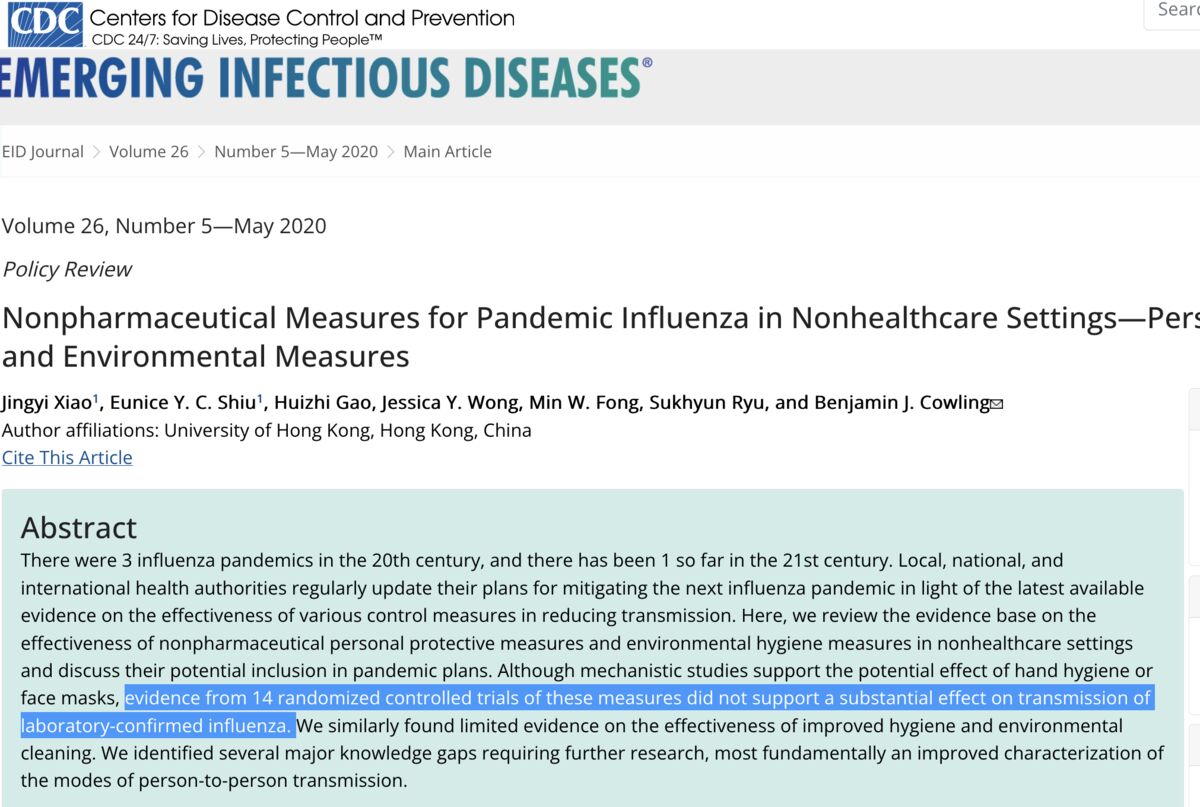Screen capture from the Centers for Disease Control and Prevention (CDC) website. The top of the image features a blue box with white text, displaying "CDC." Below this is the text "Centers for Disease Control and Prevention" in black, accompanied by the tagline "CDC 24/7: Saving Lives, Protecting People" with a trademark symbol.

A gray box follows, titled "Emerging Infectious Diseases" in blue font. Beneath this heading, in black text, reads "EID Journal, Volume 26, Number 5, May 2020, Main Article." Further down, the text repeats, specifying "Volume 26, Number 5, May 2020, Policy Review: Non-Pharmaceutical Measures for Pandemic Influenza in Non-Healthcare Settings and Environmental Measures." A list of authors is then provided, along with their affiliations: "University of Hong Kong, Hong Kong, China." 

The phrase "cite this article" appears in blue, leading to a mint-green box containing the abstract in black font. The abstract discusses the history of influenza pandemics in the 20th and 21st centuries, noting the frequent updates by health authorities to pandemic plans based on emerging evidence. The review explores the effectiveness of non-pharmaceutical personal protective measures and environmental hygiene in non-healthcare settings, aimed at controlling influenza transmission.

Key findings highlighted in blue and white text indicate that, despite mechanistic studies suggesting potential benefits of hand hygiene and face masks, evidence from 14 randomized controlled trials did not show a significant impact on the transmission of laboratory-confirmed influenza. Black text further states the limited evidence supporting the effectiveness of enhanced hygiene and environmental cleaning measures. The review identifies crucial knowledge gaps needing further research, particularly in understanding modes of person-to-person transmission.